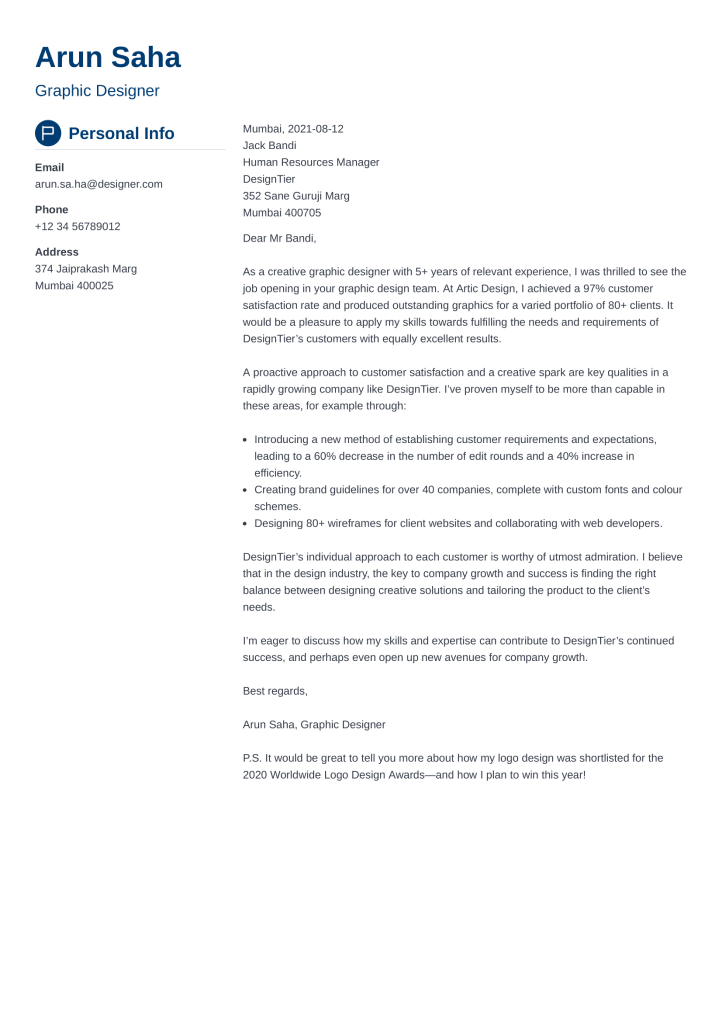**Detailed Descriptive Caption:**

The image depicts a formal letter presented on a white background, designed in portrait orientation. The letterhead prominently displays the name "Arun Saha" in bold and large dark blue font at the top left corner. Directly beneath this, in a smaller font, the title "Graphic Designer" is indicated. Following that, the section labeled "Personal Info" is headed by a dark blue circular icon with a white letter "P" inside it.

A thin horizontal line separates this header from the contact details listed below, which are also in dark blue font:
- **Email:** [Email address is provided]
- **Phone:** [Phone number is provided]
- **Address:** [Complete address in Mumbai]

The main content of the letter starts with the location "Mumbai" and is dated "2021-08-12," indicating either August 12th or December 8th, depending on the date format. Addressed to "Jack Bandy, Human Resources Manager" of an unspecified group, the letter serves as a business communication, more precisely, a job application letter.

The initial paragraph of the letter is typewritten with very small text making it difficult to read. However, it begins with the statement expressing Arun Saha's excitement about the job opening at a graphic design firm, potentially named "AI Art Design."

The content outlines Arun Saha's qualifications:
- Over 5 years of relevant experience as a creative graphic designer
- A proactive approach to customer satisfaction

The structured format includes several blank lines between sentences and a bulleted list comprising three items that possibly elaborate on specific skills or achievements.

In the concluding paragraph, Arun states: "I'm eager to discuss how my skills and expertise can contribute to Design Tiers' continued success and perhaps even open up new avenues for company growth."

The closing features "Best regards," followed by the signatory line "Arun Saha, Graphic Designer."

There is a postscript labeled "PS" but the remaining content is unreadable.